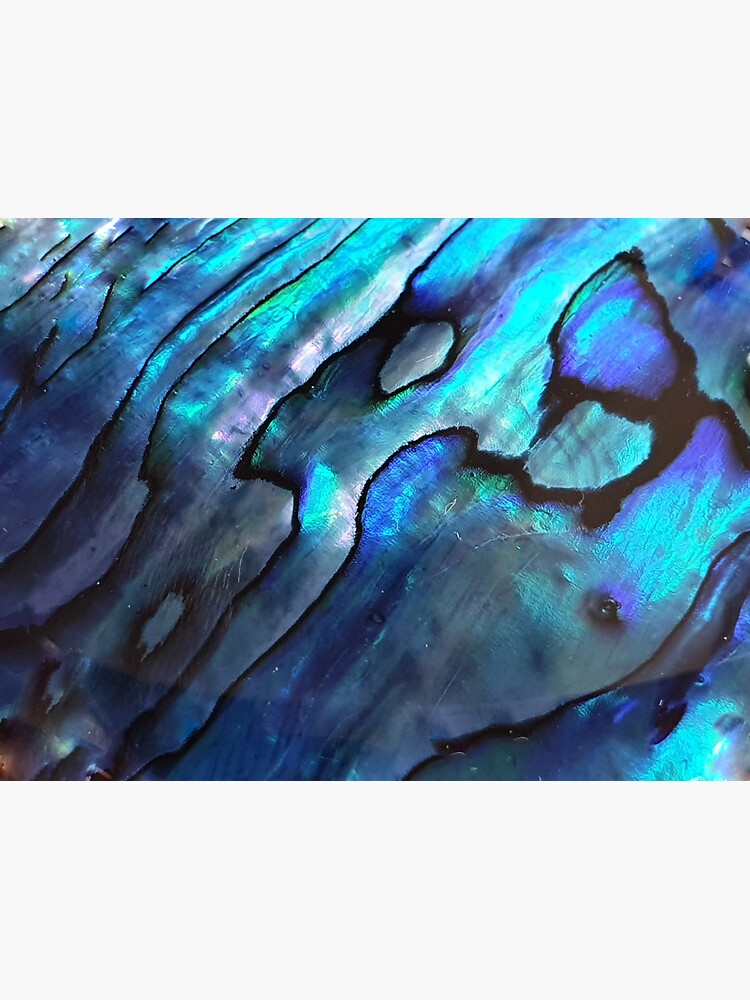The image depicts a richly textured and abstract painting that resembles a close-up view of a natural material, perhaps stone or wood, with intricate, slightly curved, and wavy lines. These lines, varying in shades of light blue, dark blue, aqua green, and hints of purples and grays, are delineated by black, almost grain-like lines, giving the impression of wood grain or stained glass. The composition is un-uniform, with horizontal rectangular orientation, and features several splotches or blotches scattered throughout. Notably, there are circular shapes and ovals, resembling knots in wood, with one prominent black knot near the center and a smaller one towards the bottom. Additional splotches vary in color and intensity, including off-white, silverish hues, and a notable darker blue near the middle. The image also reflects light, which creates lighter areas, particularly at the bottom, adding a shiny, almost luminescent quality to the intricate and layered design.